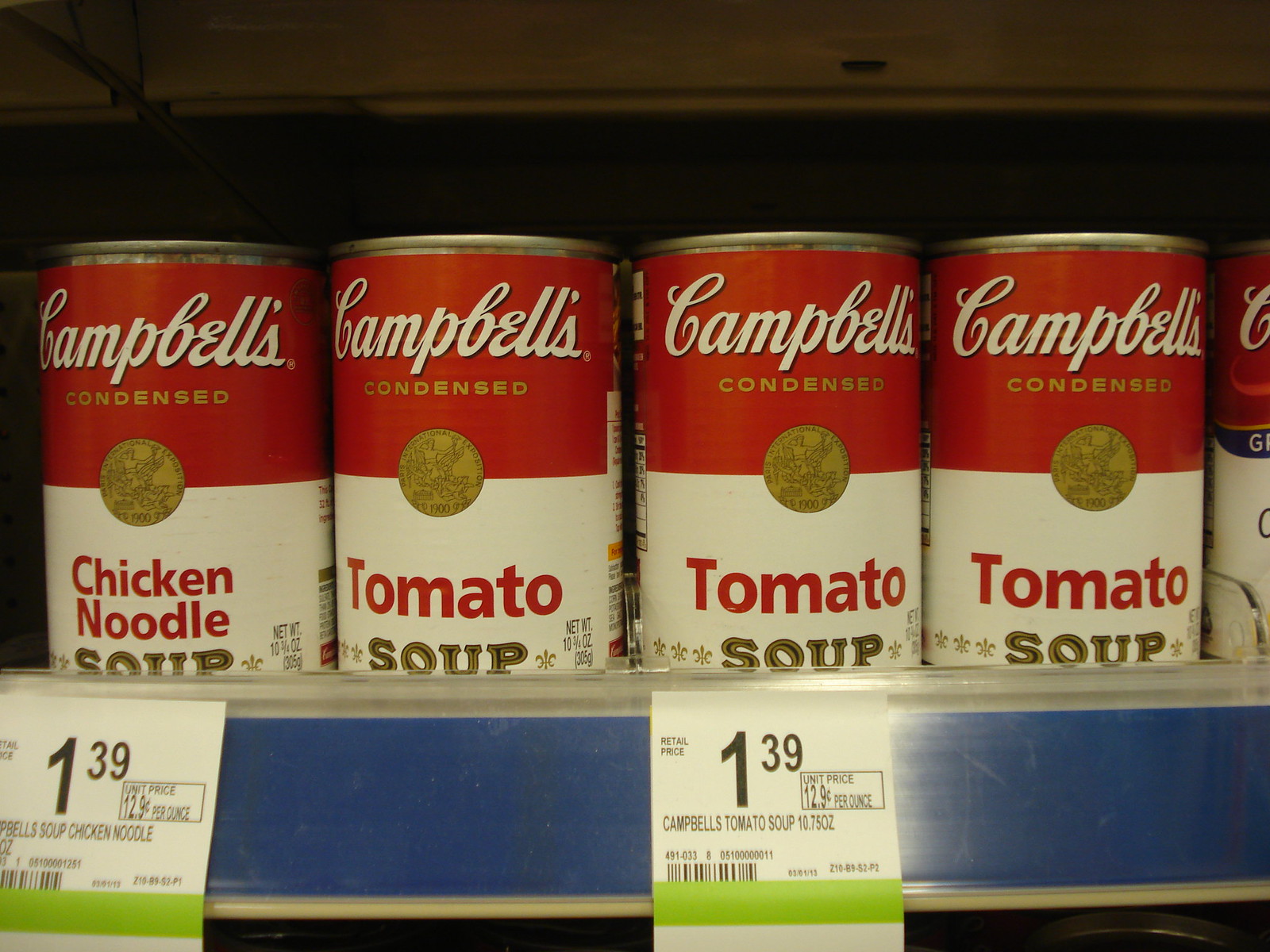This color photograph features a store shelf lined with four prominently displayed cans of Campbell's Soup, with a fifth can partially visible on the far right edge, though incomplete in view. From left to right, the visible cans are organized as follows: one can of Chicken Noodle Soup, followed by three consecutive cans of Tomato Soup. Each can's label is consistent in design, with the top section being red and showcasing the iconic Campbell's logo in elegant white script. Beneath the logo, 'Condensed' is printed in gold lettering. The lower section of the label is white, indicating the soup type in bold red letters, while the word 'Soup' appears beneath it in gold, flanked by a decorative fleur-de-lis pattern on each side. A gold circle featuring an indistinct image completes the label design. Price tags below the cans indicate that both the Chicken Noodle and Tomato soups are priced at $1.39 per can.